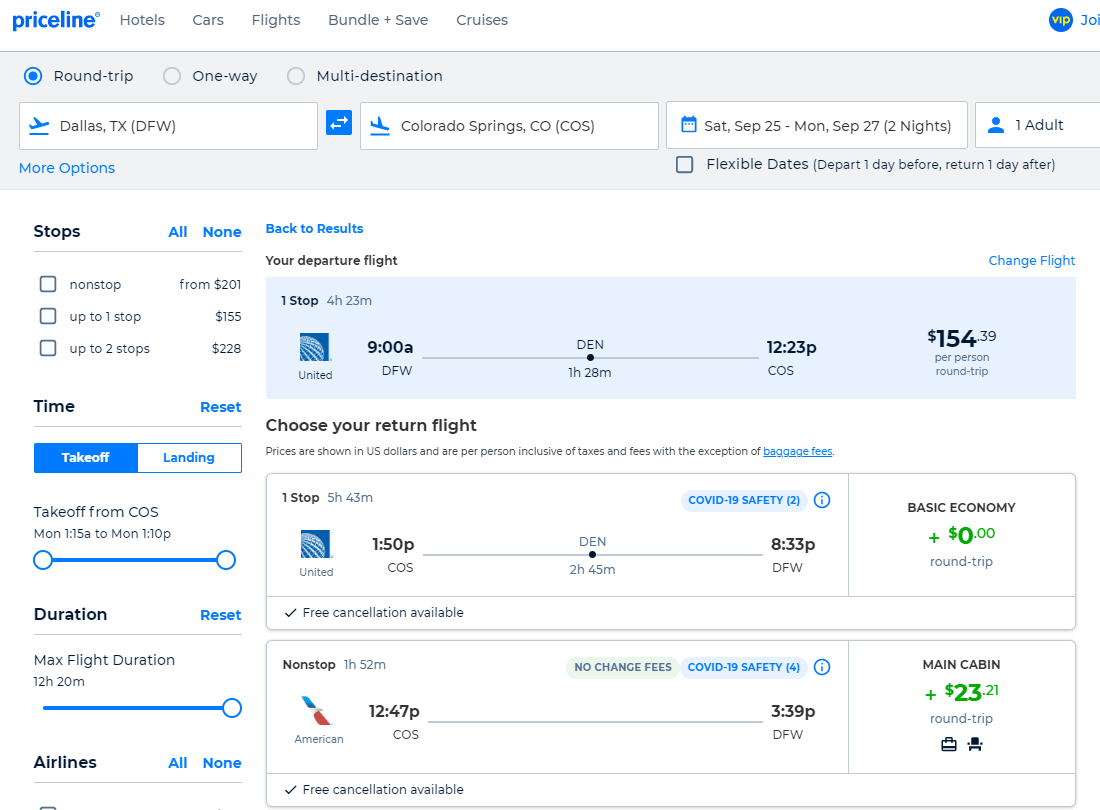Snapshot Description: Priceline Flight Booking Page

In this image, we see a snapshot taken from the website Priceline, as indicated by the Priceline logo in the top left-hand corner. The logo features the word "Priceline" in a blue font. This particular page is dedicated to booking a flight for one adult traveling from Dallas, Texas to Colorado Springs, Colorado.

The travel dates specified are a departure on Saturday, September 25th, and a return on Monday, September 27th. The body of the page provides detailed information about available flight options, including two airlines: United and American Airlines. For each airline, the page lists the flight duration, start times, and arrival times. Additionally, the flight prices are displayed, with some options priced at $154.39.

The page also highlights add-on options available at the bottom, offering various enhancements for the flight. On the left side of the screen, there are additional filtering options, allowing users to select non-stop flights or those with one or two stops. The prices for these options are listed to the right of the filters, providing a comprehensive overview of the different travel arrangements and their respective costs.